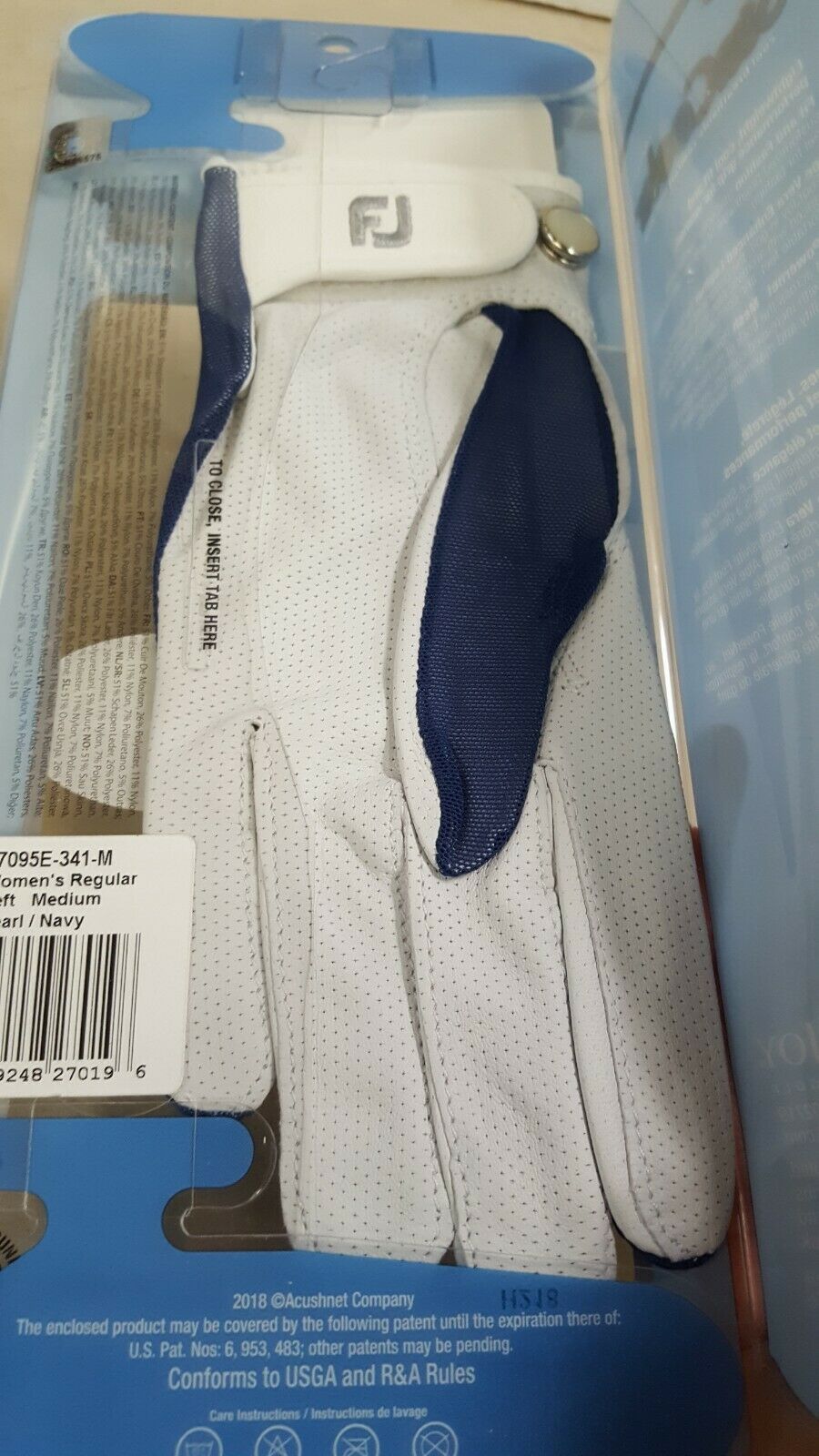The image is a detailed photograph of a golf glove, prominently featured inside its packaging. The glove itself is primarily white with a navy blue thumb and additional blue detailing on the reverse side. There is a strap around the wrist that secures with a silver snap and Velcro, and it displays the initials "FJ" in gray embroidery. The glove appears to be new and untouched, positioned within a clear packaging that reveals plenty of text, including a barcode that reads "women's regular, medium, pearl, navy color". The packaging is predominantly gray and blue, with text noting that the glove conforms to USGA and R&A rules established in 2018. The glove's material seems to be a mesh, adding to its detailed design.